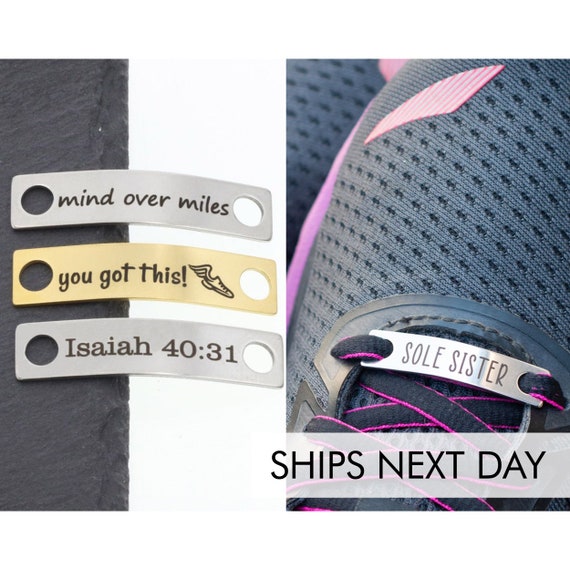The image is an advertisement presented in a split-screen format, with the left side showcasing a gray slate background adorned with three narrow, metallic badges designed for shoelaces. Each badge, rectangular with circular holes at either end, bears inspirational black text. The top silver badge reads "Mind Over Matter," the middle gold badge features "You've Got This!" accompanied by an image of a sneaker with a wing, and the bottom silver badge is inscribed with "Isaiah 40:31." The right side of the image provides a close-up view of a gray and purple sneaker with black laces trimmed in pink. Attached to the front of the laces is one of these badges, displaying "SOUL SISTER" in all capital letters. Additionally, the phrase "Ships Next Day" appears in black text at the bottom right corner of the image, all displayed in a sans serif font.